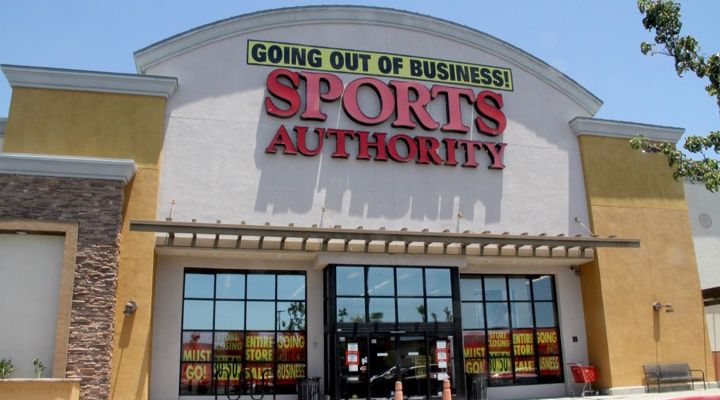This image features the storefront of a Sports Authority store. Dominating the scene is a prominent yellow rectangle sign at the top, emblazoned with "GOING OUT OF BUSINESS" in bold black letters. Just below it, "Sports Authority" is displayed in striking red letters. The storefront is framed by two yellow rectangular pillars, and the top of the building features an arch set against an off-white beige backdrop. 

At ground level, the entrance consists of four large doors flanked by clean, reflective windows arranged in four-by-four squares. These windows are adorned with red signs bearing bold yellow lettering that declare, "MUST GO - ENTIRE STORE - GOING OUT OF BUSINESS," along with promotional messages like "STORE CLOSING" and "30 TO 50% OFF." 

On the right side of the entrance, a lone red shopping cart is positioned in the corner, and adjacent to it, a gray bench with a light fixture overhead provides a resting spot for shoppers. Near the doors, two yellow cones or trays are placed, enhancing the sense of a store in its final days of operation.